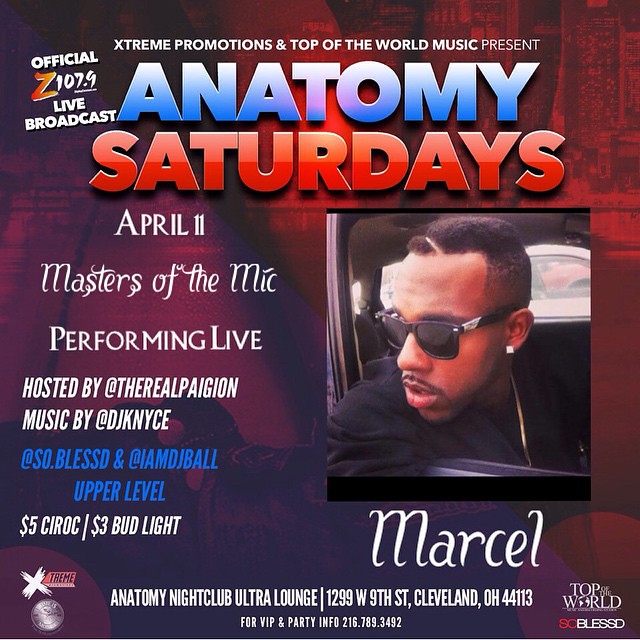The poster advertises a vibrant event titled "Anatomy Saturdays," organized by XTREME Promotions and Top of the World Music. The background transitions from purplish hues on the left to reddish-brown on the right, featuring textured city skyline elements.

At the top, small white text announces the organizers. Prominently displayed in bold, "Anatomy" appears in blue and white lettering, while "Saturdays" is in red. To the left, a smaller text notes “Official Z 107.9 Live Broadcast,” with the station's logo in a blend of orange and yellow.

Below, in white font, the date "April 11th" is stated, followed by the event tagline, "Masters of the Mic," in a cursive italic font. Subsequently, it mentions "Performing Live" and "Hosted by The Real Pagan," with music by "DJ Nice." There's also mention of social media handles, “@SoBlessed” and “@IAmDJBall.”

An eye-catching photograph of an African American man leaning out of a car window is featured on the right. He sports dark sunglasses, a diamond stud earring, short hair with a line pattern, a thin mustache, a light beard, a black shirt, and a gold chain. Below this image, the name "Marcell" is highlighted in large white text.

Further down, the venue details are provided: "Anatomy Nightclub Ultra Lounge" at "1299 W 9th Street, Cleveland, Ohio 44113," along with a contact number for VIP and party information, "216-789-3492."

At the bottom, various logos are present, including "EXTREME" in a combination of white and black, and "Top of the World" in red and white. Another logo "So Blessed" is also visible, with "So" in red and "Blessed" in white. The entire vibrant composition directs viewers' attention towards an exciting and well-organized event.